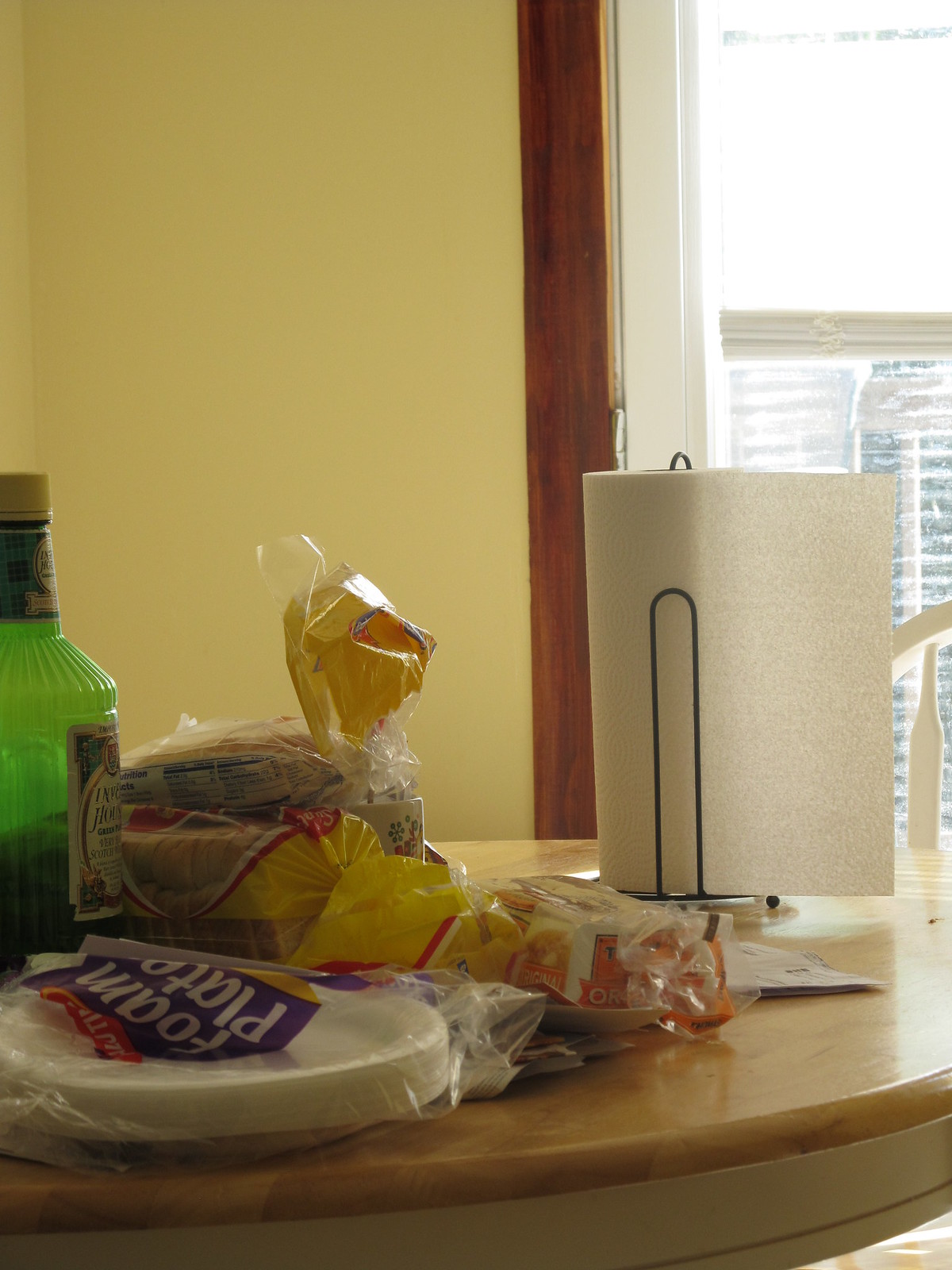This image captures a bright, inviting kitchen bathed in natural light. The walls, painted a soft, warm yellow, frame a cozy, lived-in space. Wooden trim in a rich brown color encircles the window, adding a touch of rustic charm. A round table commands attention at the center of the room, with a smooth wooden top and a cream-colored base adorned with a subtle gold stripe. Matching chairs surround the table, featuring white rungs that maintain the room’s airy feel.

On the table, a few everyday items bring the scene to life. A silver and black paper towel dispenser stands ready with a roll of paper towels, its wire hook design allowing for easy tearing. Nearby, a plastic bag with vibrant red and yellow accents suggests it contains a loaf of bread. A clear package marked “Foam Plates” sits next to it, reinforcing the sense of practicality. In the background, a green bottle with a white cap—possibly vinegar or alcohol—adds a touch of color, its label featuring details around the neck and front.

Overall, the image conveys a warm, functional kitchen, harmonizing bright colors and natural materials in a welcoming domestic setting.